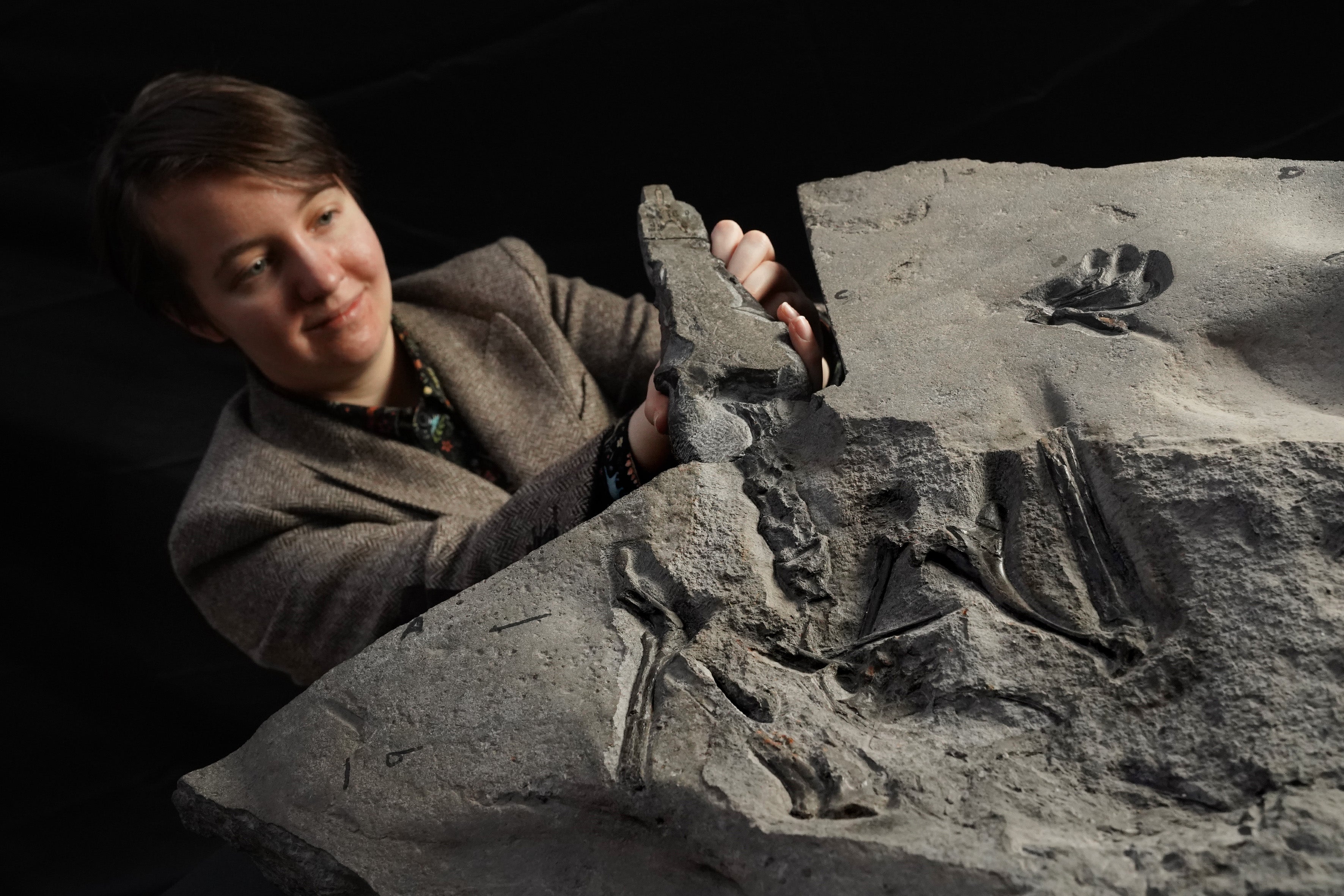A high-quality color photograph features a large, jagged rock with various indents and a flat section at its center, possibly bearing ancient footprints or hieroglyphics. The rock's surface, predominantly gray and rugged, shows intricate carvings or natural imprints, notably a paw or hand print at the top right. On the left side of the image stands a young individual, approximately 18 years old, with short, slightly parted hair, seemingly focused and exhibiting a slight smile. This person is dressed in a gray tweed sport jacket over a patterned shirt that suggests a planetary design. They have their hands on the edge of the rock, which is set against a solid black backdrop, and there are no other people or legible inscriptions visible in the photograph.